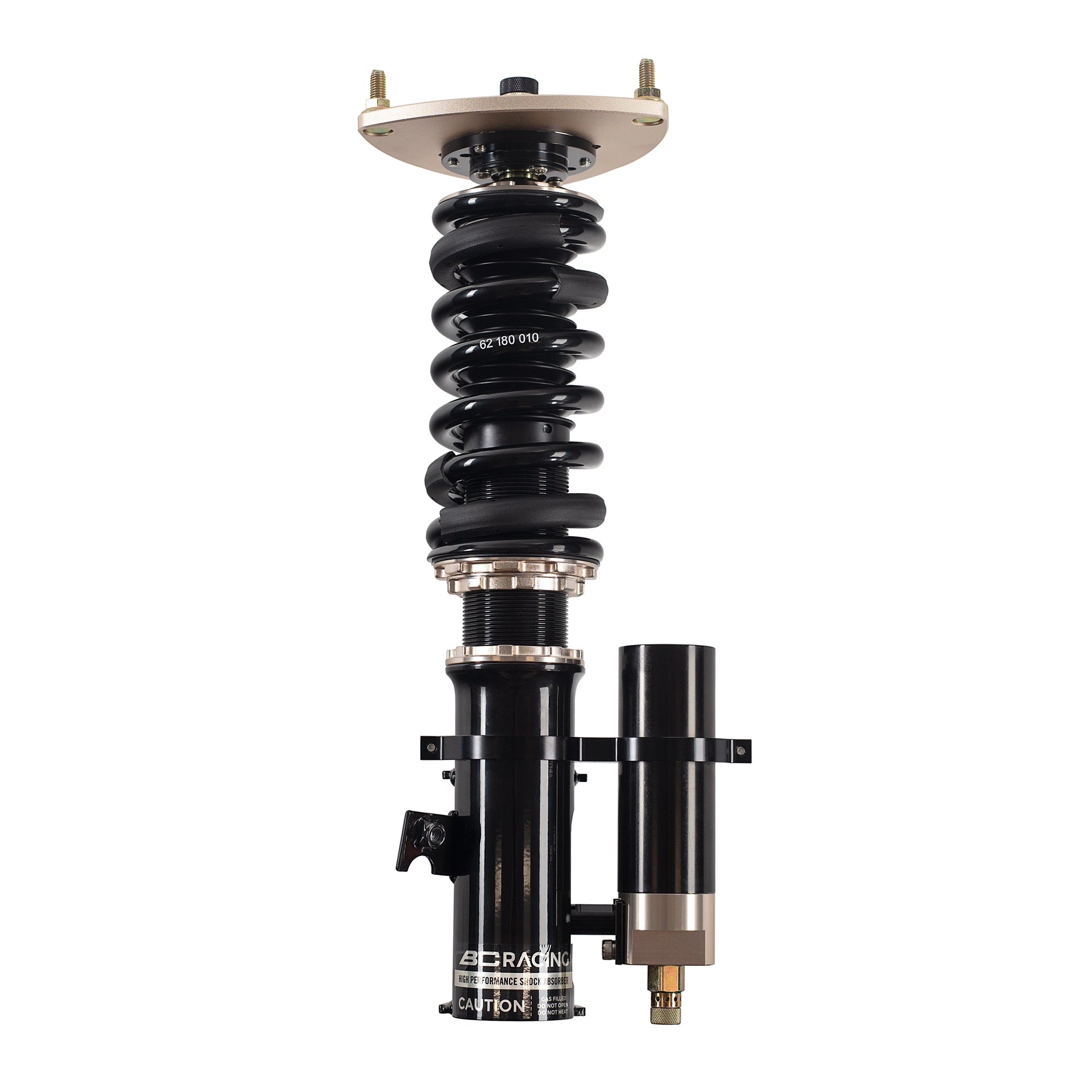This color photograph, set against a white background, depicts a high-performance shock absorber. At the top, a brushed silver metal mount is securely fastened with screws, creating a triangular pattern. Immediately below, a black threaded rod runs through the assembly, wrapped with a shiny, black spring-like coil. In the middle of this coil, white numbers "6218010" stand out prominently. The device transitions into a glossy black cylinder that features the cautionary label "BC Racing High Performance Shock Absorber" at the bottom, although the exact cautionary details are not legible. Adjacent to this cylinder, another smaller black cylinder is connected, adding complexity to the overall structure. The various polished and glossy surfaces on the device reflect light, highlighting its industrial design and intricate details.